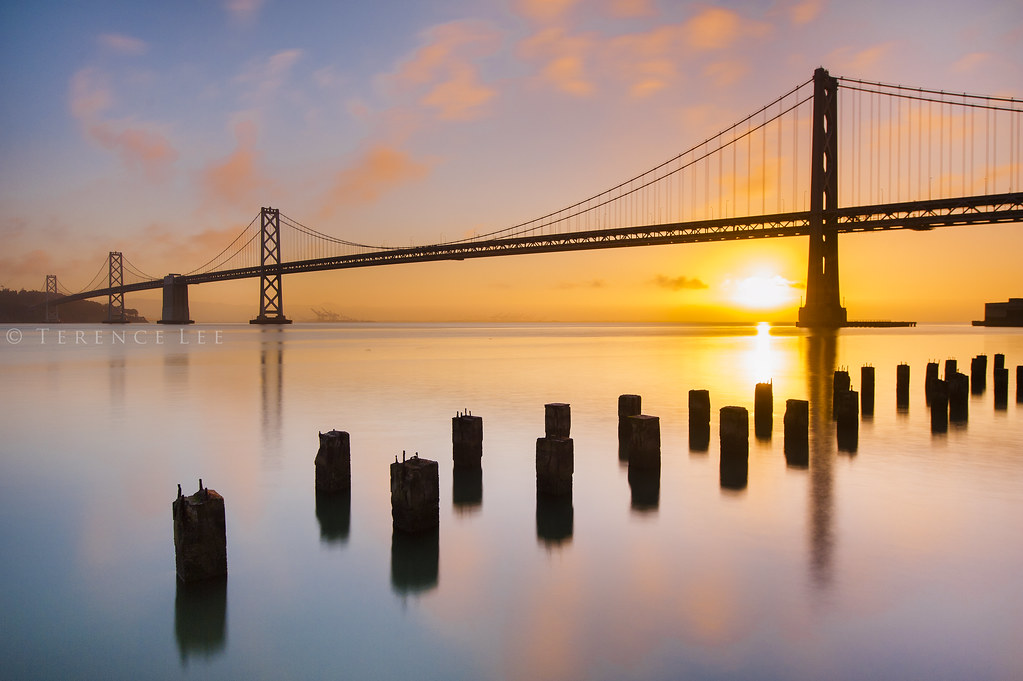This captivating photograph, taken by Terrence Lee, features the San Francisco Bay Bridge at either sunrise or sunset, offering a striking interplay of light and color. The suspension bridge elegantly spans the center of the image, with the sun in the background casting vibrant red, orange, peach, and yellow hues across the sky and water. Captured from a water-level perspective, the bridge appears to recede into the distance towards the left, with its nearest tower prominently closer to the observer. Below, calm bay waters reflect not only the sun but also the intricate details of the bridge and its surroundings, enhancing the photo's evocative nature. 

In the foreground, wooden pier supports punctuated with metal spikes rise from the water, leading the eye diagonally from the lower left towards the middle right of the image. Behind these piers, delicate fog partially shrouds the bay, adding to the mood of the scene. The sky above is adorned with blue tones and cotton ball-like pink clouds, painting a serene backdrop. The minimal horizon captures the last rays of sunlight, a bright orb positioned near the first pier on the left. The photographer's name, Terrence Lee, is subtly inscribed in white along the middle of the left-hand border, marking this exquisite and evocative composition.